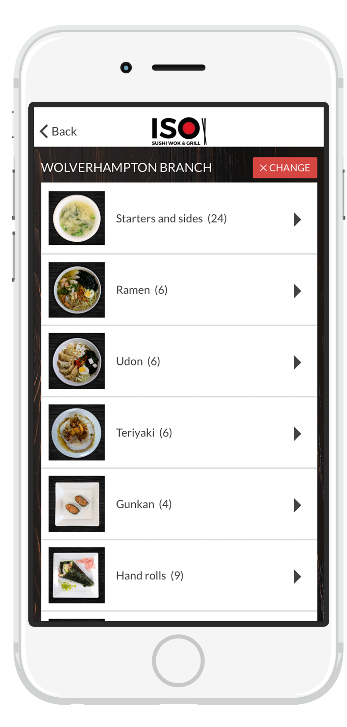The image is a vertical rectangle featuring a smartphone displaying an app interface. The phone's frame is visible, encompassing a screen showing what appears to be a menu from a restaurant app named "ISO Sushi Walk and Grill." The restaurant's name is prominently displayed in black text on a white banner at the center of the screen, while the rest of the app background is black. Below the restaurant's name, a vertical list of menu categories is displayed, each accompanied by an image on the left, a description in the center, and a forward arrow button on the right.

The menu categories are as follows:
- Starters and Sides (24 items)
- Ramen (6 options)
- Udon (6 options)
- Teriyaki (6 options)
- Gun Ken (4 options)
- Hand Rolls (9 options)

At the top of the menu list, there is text indicating the "Wolverhampton Branch" of the restaurant, with a red "Change" button to the right, allowing users to change the location.